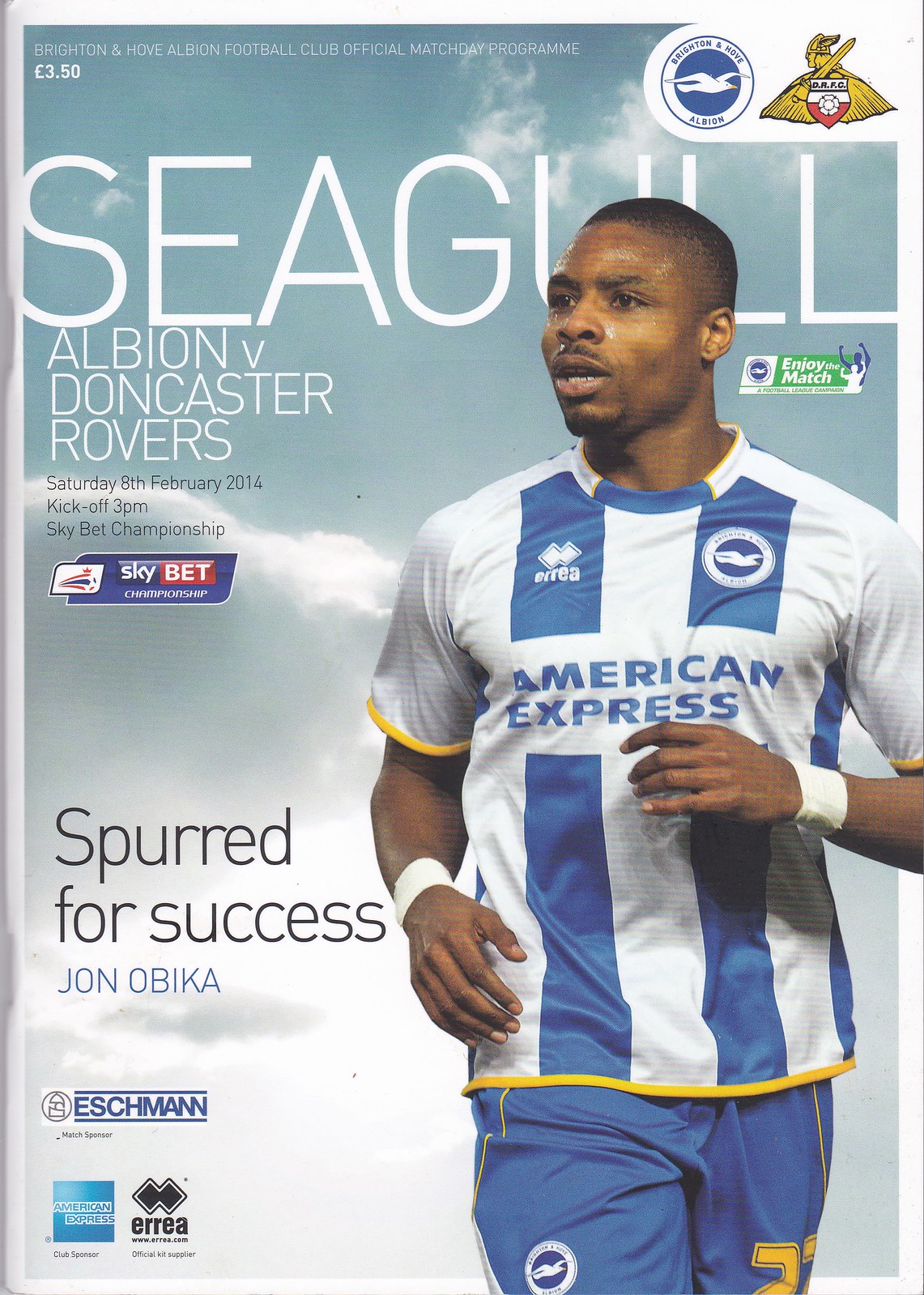This is a detailed magazine cover for a soccer team. The title "Seagull" is prominently displayed in large white font at the top, partially obscured by the head of a sports player on the right, who is dressed in a white and blue shirt with "American Express" written on it, as well as matching blue shorts. The player also sports white wristbands with yellow stripes and has a number in yellow on his shorts, although only the top of the number is visible.

The background features a blue sky with white and gray clouds. Below the title on the left side of the cover, it reads: "Albion vs. Doncaster Rovers, Saturday, 8th February, 2014, kick-off, 3 p.m., SkyBet Championship." Beneath this, there's the SkyBet logo followed by the text "Spurred for Success, Joan Obika, Eschmann."

In the bottom left corner, there are two logos, one for American Express and another for El Río, with additional logos present in the top right corner of the image.